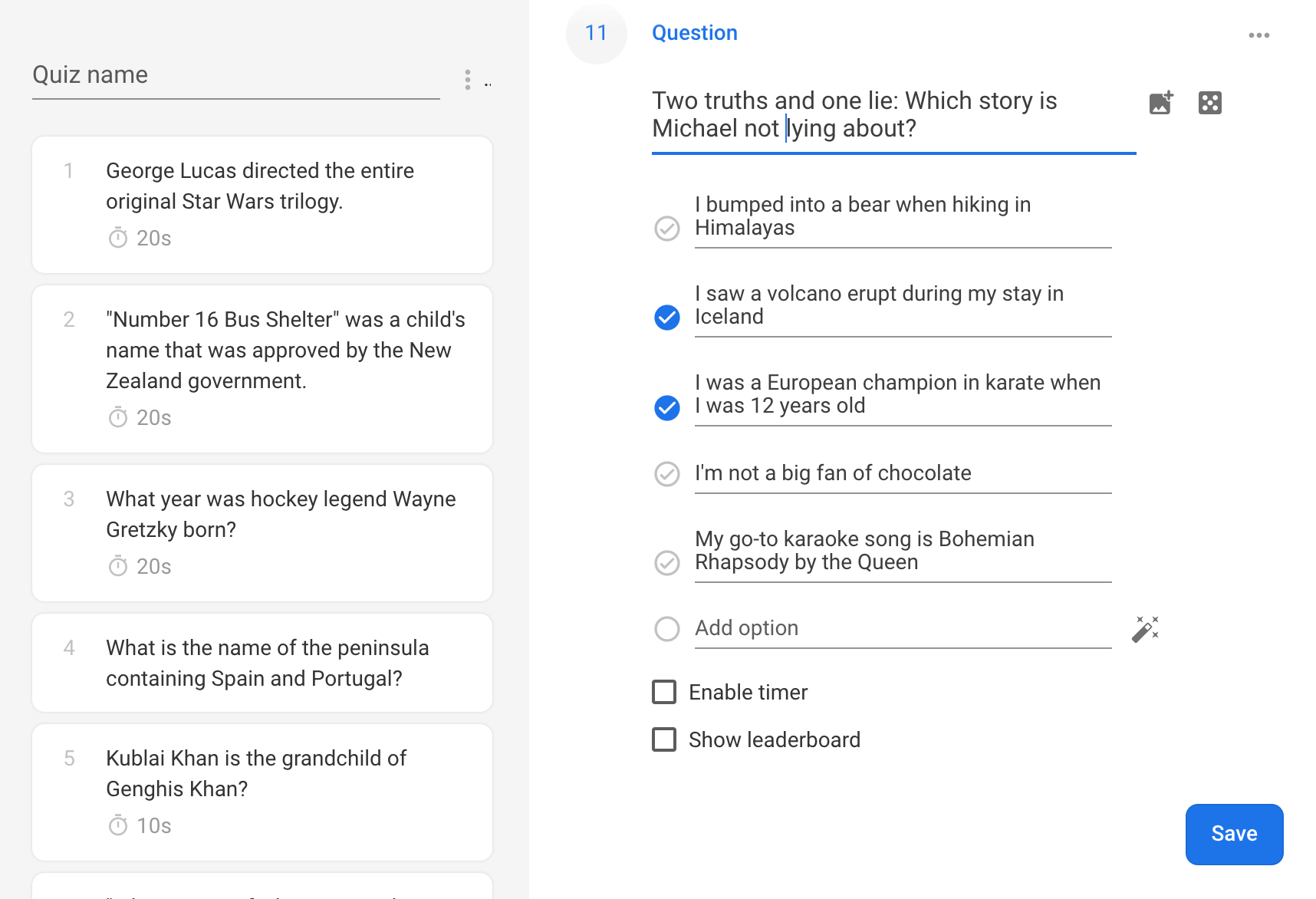In the provided image, there are two adjacent sections, each resembling columns. The left section is distinctly highlighted in a lilac background, whereas the right section is primarily in white and black with accents of blue. These sections function as separate posts rather than traditional columns.

The left section, titled "Quiz Name," lists five quizzes with various labels. Notably, there is a listing where "George Lucas directed the entire original Star Wars trilogy" is shown with a time mark of 20 seconds. Another notable entry is quiz number 16, labeled "Bus Shelter," which intriguingly states that this was a child's name approved by the New Zealand government.

In contrast, the right section is titled "Two Truths and One Lie." It poses the challenge, "Which story is Michael not lying about?" Three statements follow: "I bumped into a bear when hiking in the Himalayas," "I saw a volcano erupt during my stay in Iceland," and "I was a European champion in karate when I was 12 years old." Below these statements, there is an option to add additional choices.

At the bottom of the right section, users are provided with interactive options, including "Enable Timer" and "Show Leaderboard." There is also a save button to preserve changes.